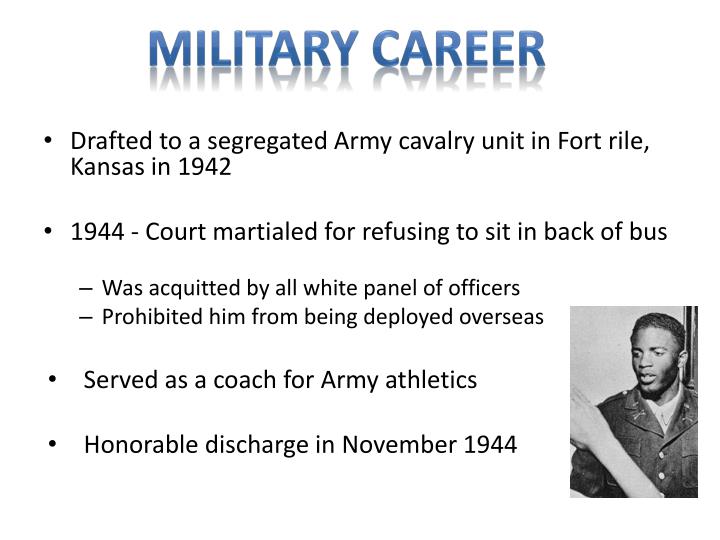The image depicts a PowerPoint slide titled "MILITARY CAREER" in stylized, medium blue, capitalized letters with a gray shadow effect. Below the title are several bullet points detailing key events: 

1. Drafted to a segregated Army cavalry unit in Fort Ryle, Kansas, in 1942.
2. In 1944, court-martialed for refusing to sit at the back of the bus, acquitted by an all-white panel of officers, and prohibited from being deployed overseas.
3. Served as a coach for Army athletics.
4. Received an honorable discharge in November 1944.

In the lower right corner of the slide, there is a small rectangular black-and-white photograph of a man in Army attire, facing to the left, presumed to be the subject of the slide. The background of the slide is plain white, highlighting the text and image.